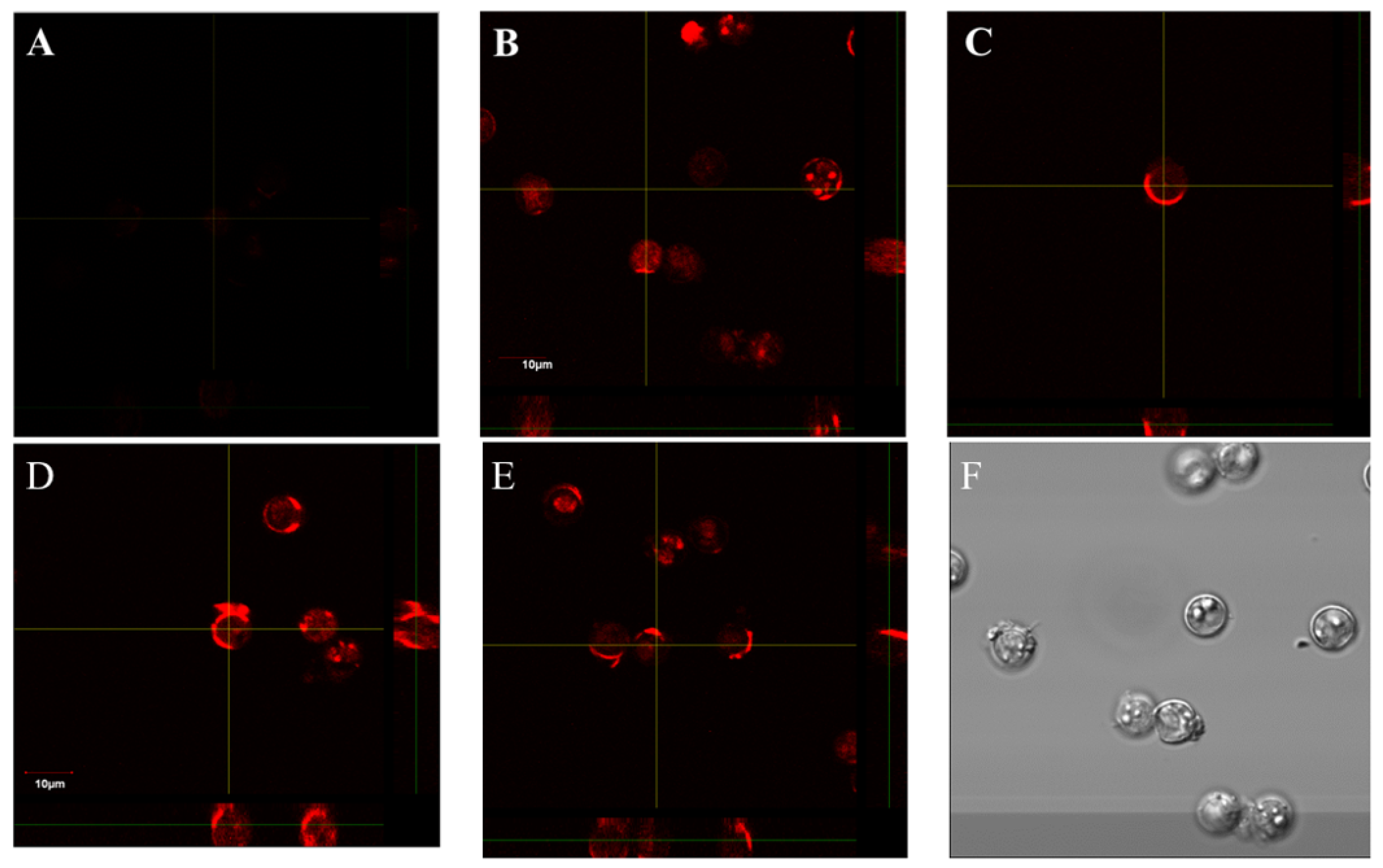The image is a horizontally arranged scientific notification chart composed of six square quadrants labeled A through F. In the top row are A (far left), B (middle), and C (far right), and in the bottom row are D (far left), E (middle), and F (far right). 

- Quadrant A is entirely black with a crosshair in the center.
- Quadrants B through E feature a black background with red, glowing, neon-like circular objects. Each has a crosshair in the center targeting these red circles. Specifically:
  - B has scattered red circular objects.
  - C has a prominent red circle at the crosshair. 
  - D shows multiple red circles with one centered on the crosshair and features a label that reads "10" in the lower left.
  - E displays numerous red circles with a focus on one at the crosshair, and several others scattered around.
- Quadrant F deviates significantly with a gray background and small, clear, bubble-like structures, some of which are clumped together.

The entire image looks like a scientific study, possibly showing microscope views focusing on red fluorescent objects and features a mix of grayscale and color-coded elements to differentiate the specimen types.